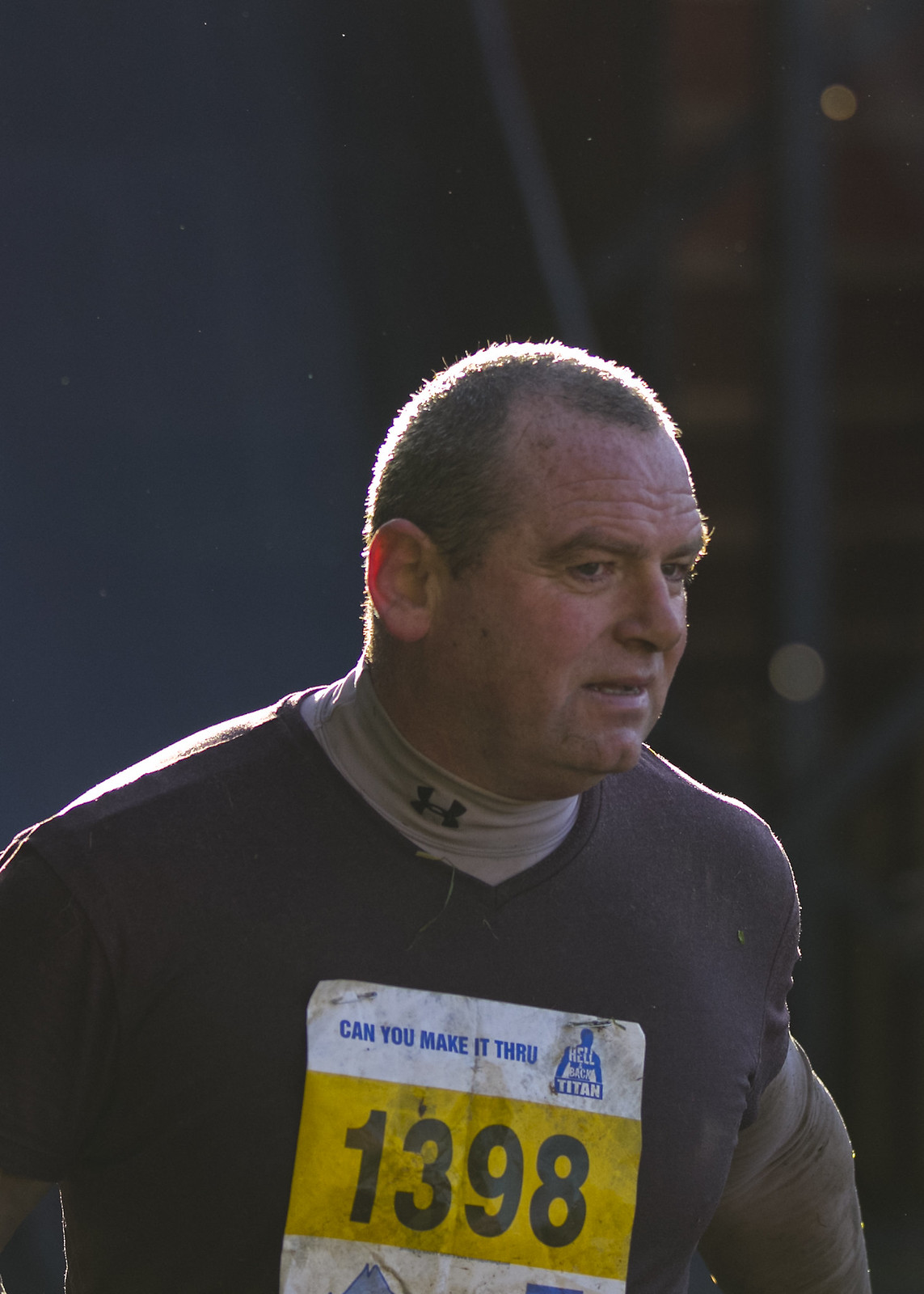This photo features an older white man participating in a marathon, as indicated by the race number 1398 emblazoned on a yellow caution-colored backdrop pinned to his brown shirt. The man, who looks quite fit for his age, is wearing a tan Under Armour turtleneck undershirt with a black logo on the collar, visible beneath his brown shirt. The shirt bears the inscription "Can you make it through?" followed by the word "Titan" and a small blue figure, all printed in blue text on a white backdrop. The man appears to be looking slightly away from the camera, and the photo captures a moment of sunlight shining on his head, creating a contrast with the darker area in front of him. The background includes a red brick post with tan caulk and a blue area on the wall, alongside a silver or blue frame. This candid shot seems to be a standard race photo taken during the event.